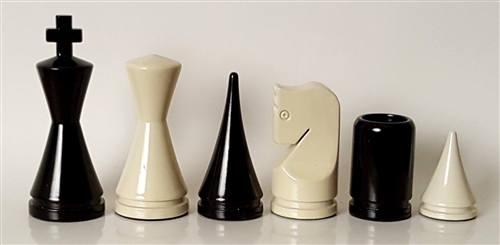The image features six chess pieces arranged in a line against a white or very light beige background. The pieces alternate in color from black to white, starting with black on the left. The set includes a black king with a cross at the top, a white queen without any top adornment, a black bishop with a triangular shape, and a white knight with a simplistic horse head. Following these are a black rook, resembling a cylinder, and a tiny white pawn with a triangular shape. The pieces are made from a shiny material, possibly plastic, acrylic, or resin, and have a modern, minimalistic design with very little detail except for the knight. The overall composition highlights the sleek and contemporary aspect of the chess pieces.